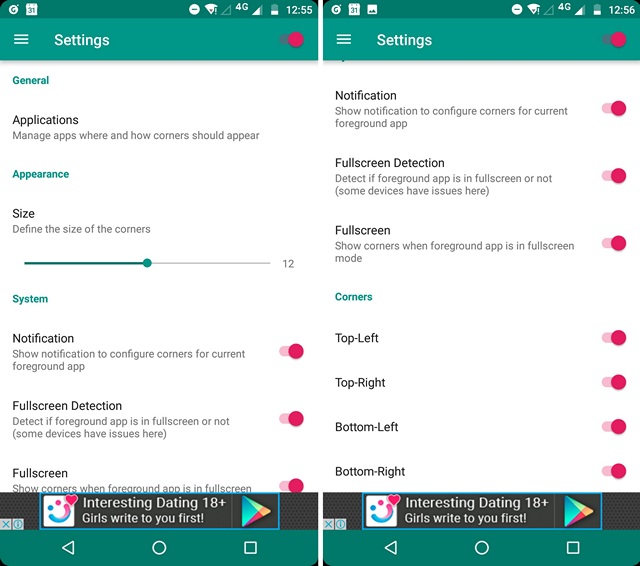These images depict two screenshots side by side from an Android device, specifically from an app's settings page. Both screenshots display the status bar at the top, featuring the Google logo, the date marked as the 31st, an exclamation point next to the Wi-Fi symbol, a 4G symbol, a battery level below 50%, and the times 12:55 PM on the left and 12:56 PM on the right.

The app's interface showcases turquoise-colored menu bars at both the top and bottom. A prominent pink circular button is situated at the top right corner of each screenshot. The left screenshot lists several menu options under "General Applications," including Appearance, Size, System Notification, Full Screen Detection, and Full Screen. An advertisement runs along the bottom, promoting "interesting dating 18+ girls write to you first."

At the very bottom, the turquoise navigation menu features three icons: a left-facing back arrow, a circle, and a square.

The right screenshot continues from where the left ends, displaying options such as Notification, Full Screen Detection, Full Screen, and settings for "Corners" (Top Left, Top Right, Bottom Left, and Bottom Right). Most options come with toggles on their right, set to "On" and depicted as pink circles. The background across both screenshots is white, with black text for the app's settings.

Overall, the screenshots provide a comprehensive look at the app's settings, highlighting both general and specific customization options.